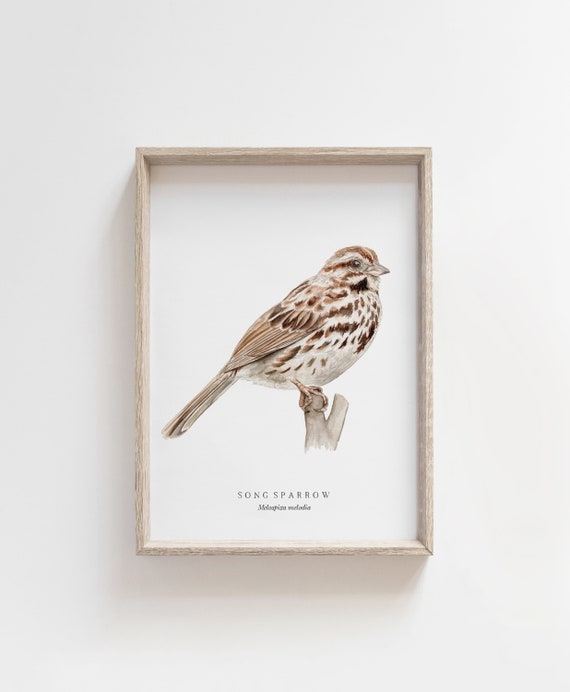The image depicts a detailed painting of a small Song Sparrow, centrally framed on a stark white background. The frame is a subtle, light grayish-brown wood, adding a simple yet natural touch to the artwork. The sparrow, perched delicately on the tip of a grayish branch, features distinct brown stripes, with brown wings, pin feathers, and a tail, along with a white underbelly adorned with brown spots. It has a brown beak, brown eyes, and a brown stripe running down its head. The bird is facing right, with its tail angled towards the bottom left corner of the painting. Below the elegantly rendered bird, the text "Song Sparrow" is inscribed, followed by what seems to be its Latin name in smaller, less readable script. This painting stands out prominently against the plain white wall, giving the impression of being showcased in a museum.